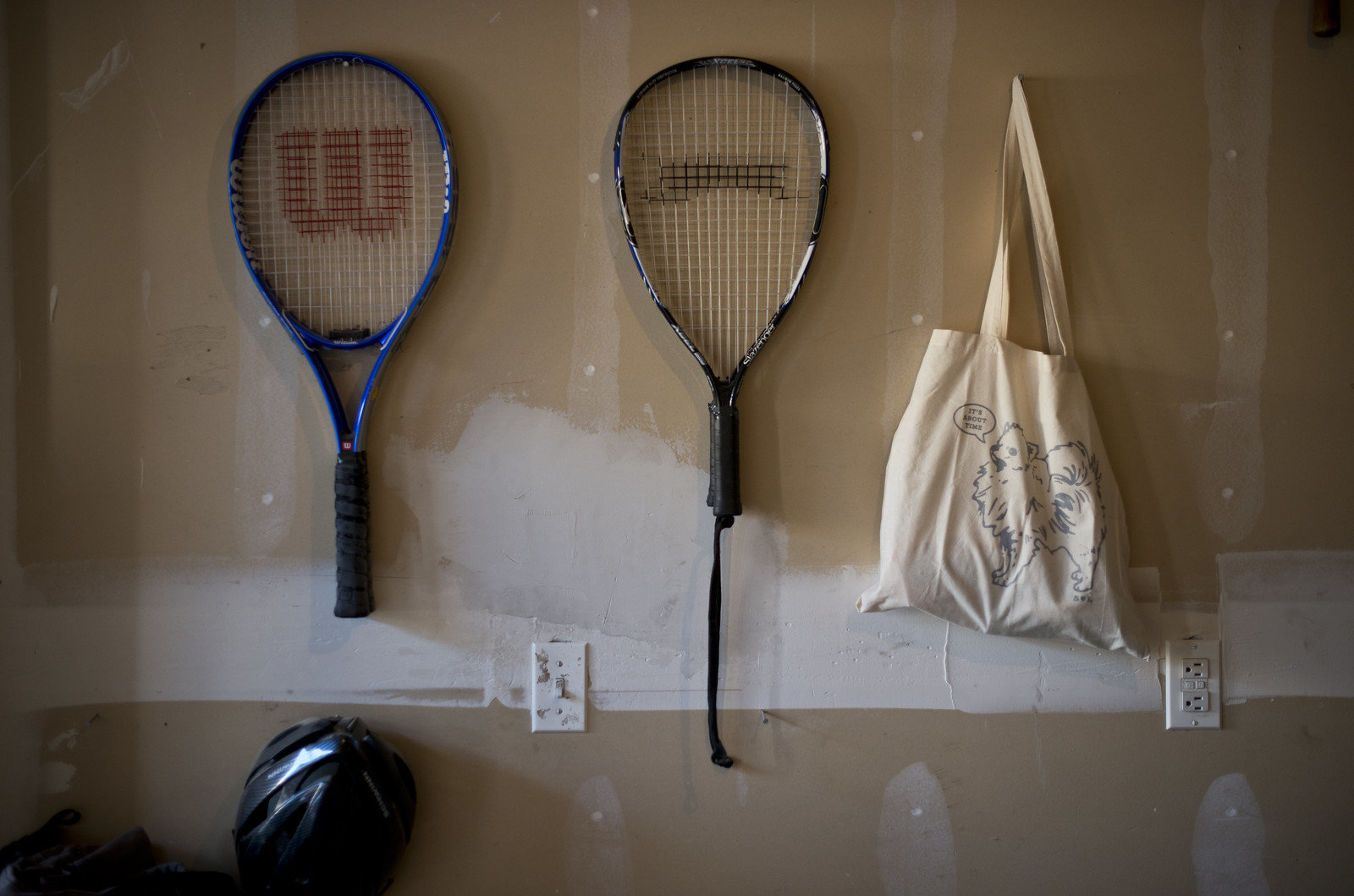The image depicts an unfinished drywall wall inside a building, possibly a garage or a sports room. The wall is roughly taped and plastered, with some plaster on a light switch and electrical socket, both white, situated between two hanging rackets. On the left side is a blue Wilson tennis racket with a brown "W" on its strings. To its right is a black and white racquetball racket with a black handle and strap hanging down. Adjacent to the racquetball racket is a cream-colored canvas tote bag featuring a black outline drawing of a Pomeranian puppy with a speech bubble saying "it's about time." Natural light highlights the tote bag. At the bottom left of the wall sits a black bicycle helmet. The overall image has a sepia tone, emphasizing colors like blue, black, cream, white, and off-white.